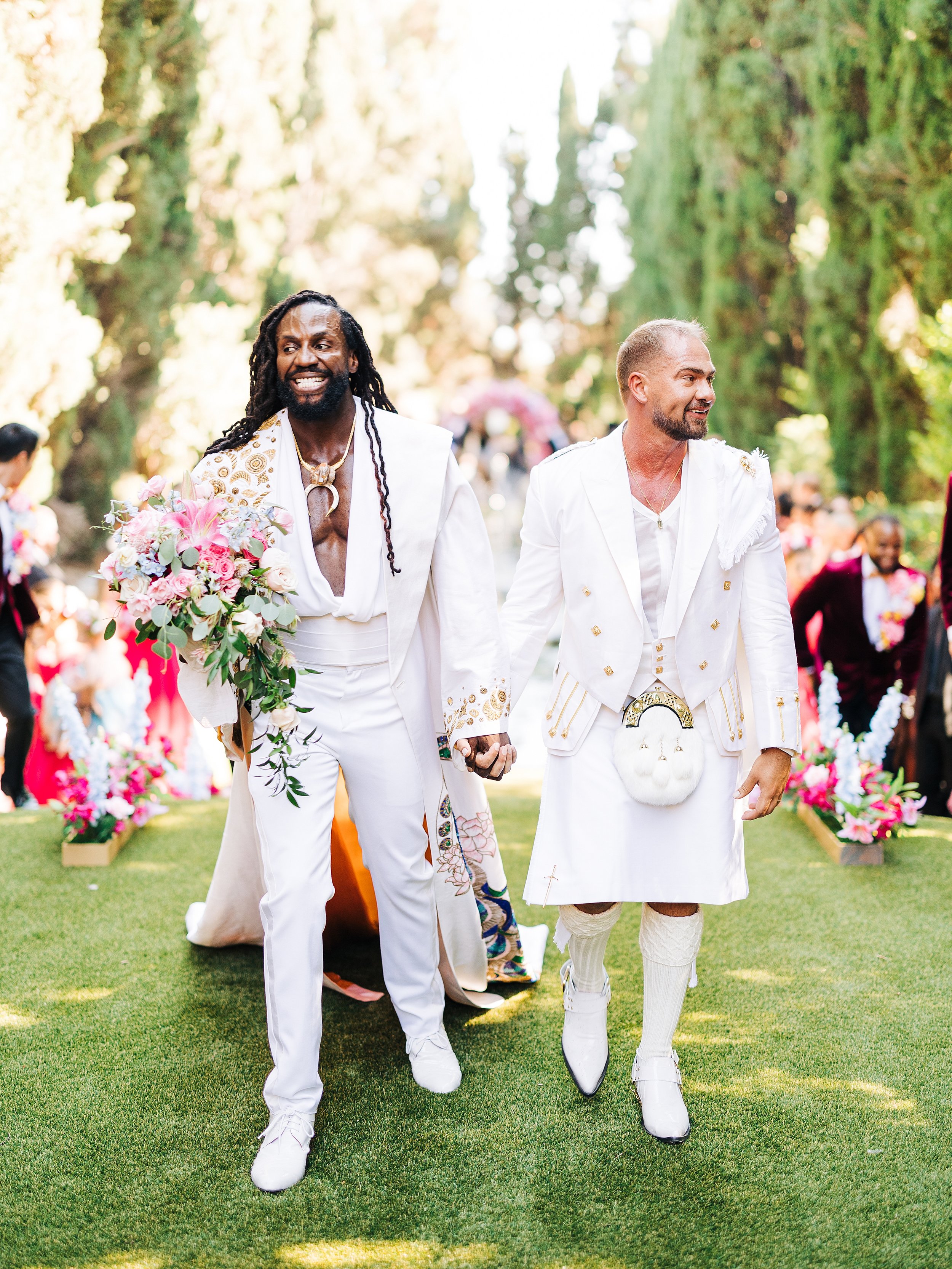In this vibrant outdoor wedding scene, two men, an interracial gay couple, are walking hand in hand down a grassy aisle surrounded by lush greenery and wedding guests. Both men are dressed elegantly in white, emphasizing the festive and joyful atmosphere. One, an African American man with long dreadlocks, wears a sharp white suit accented with a gold chain and white shoes, carrying a bouquet of pink flowers and green leaves. Beside him, a Caucasian man with blonde hair and a beard dons a white suit jacket paired with a kilt and knee-high boots, adding unique flair to his attire. The wedding guests on either side of the aisle are dressed up, some donning bright colors like pink, while others opt for more subdued hues like black. They watch with smiles as the couple, beaming with happiness, make their way down the aisle under the canopy of verdant trees.